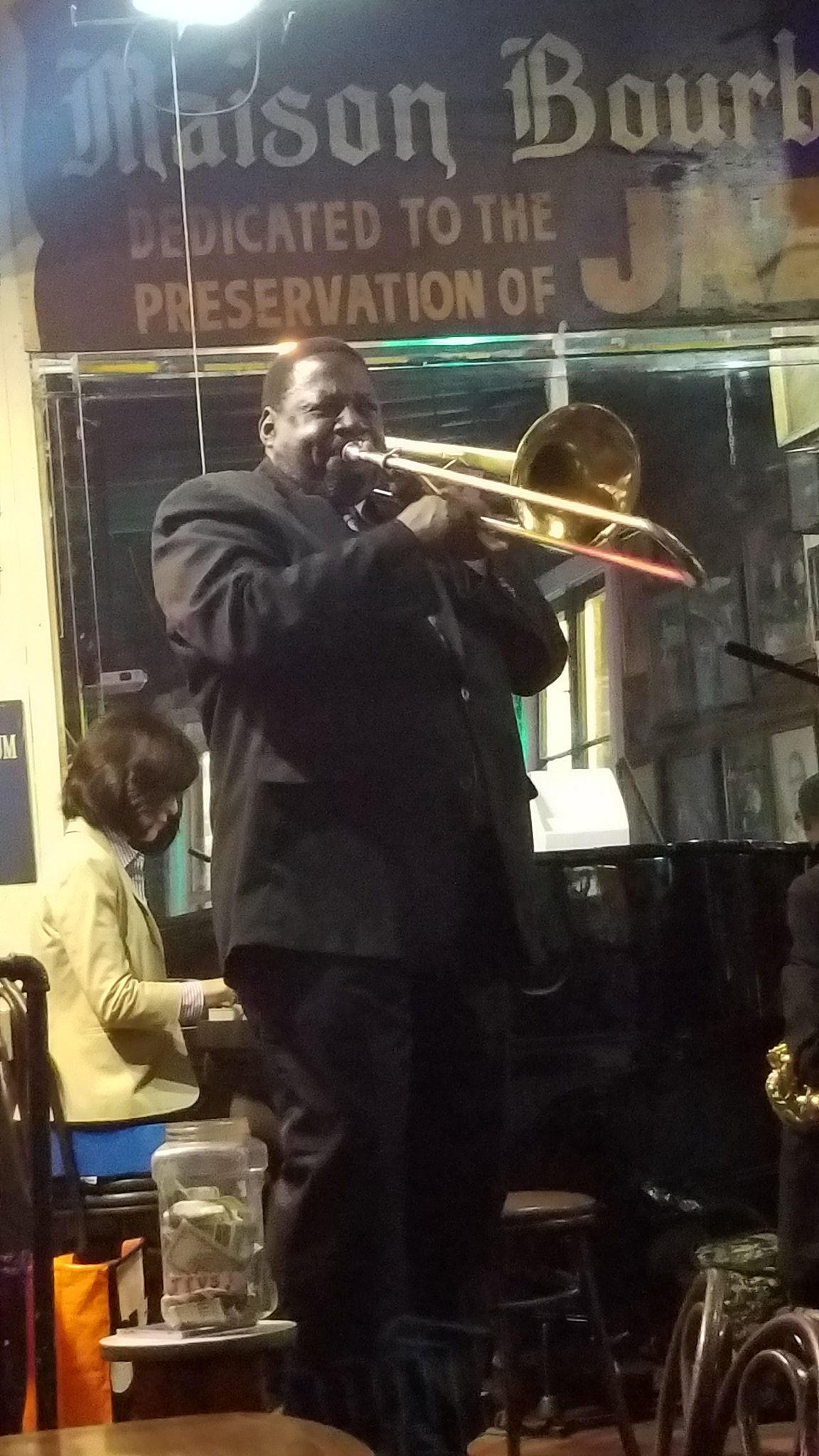A detailed image captures a bustling New Orleans jazz scene on Bourbon Street. Dominating the foreground is a heavyset, or rather obese, black man dressed in a buttoned-up black suit, complete with a tie, energetically playing a golden trombone. His focused performance takes place under a prominent sign with a red background that reads "Maison Bourbon" and a yellow subtitle declaring "dedicated to the preservation of jazz." A tip jar brimming with cash sits beside him, indicating generous contributions from the audience.

Behind him, a woman with shoulder-length dark hair, clad in a yellow jacket and blue pants, is immersed in playing the piano. The background features framed photos adorning the wall and a window that seems to extend inside the building, adding depth to the scene. Wooden tables and chairs, some possibly topped with leather, are scattered around, adding to the lively atmosphere of a quintessential New Orleans jazz venue.